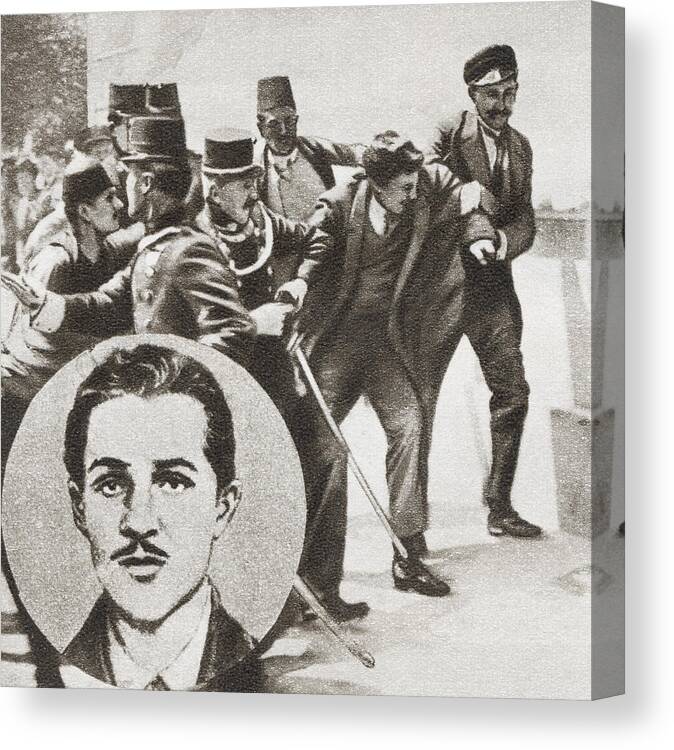This is a detailed black and white photograph of a vintage painting, printed onto a sturdy canvas without a frame, allowing the image to wrap around the edges. The scene appears to depict a historical event, potentially from the pre-World War I era or during the time of the Ottoman Empire. The central figure is a man in a suit, wearing a long overcoat and black shoes, with noticeable short curly hair and a thin mustache.

He is being forcefully apprehended by several individuals in police or military uniforms, characterized by their tall, squared-off hats and wielding swords. They are firmly grasping his arms and hands, possibly seizing a sword he holds. Behind them, more individuals in various hats and attire suggest a commotion or scuffle, with some wearing suits and top hats adding to the chaotic scene.

In the lower left corner of the painting, a large circular inset provides a detailed portrait of the apprehended man, highlighting his facial features, including dark eyebrows and a small mustache. The entire composition, done in grayscale, is reminiscent of a vintage newspaper illustration, capturing a moment of dramatic tension and historical significance.